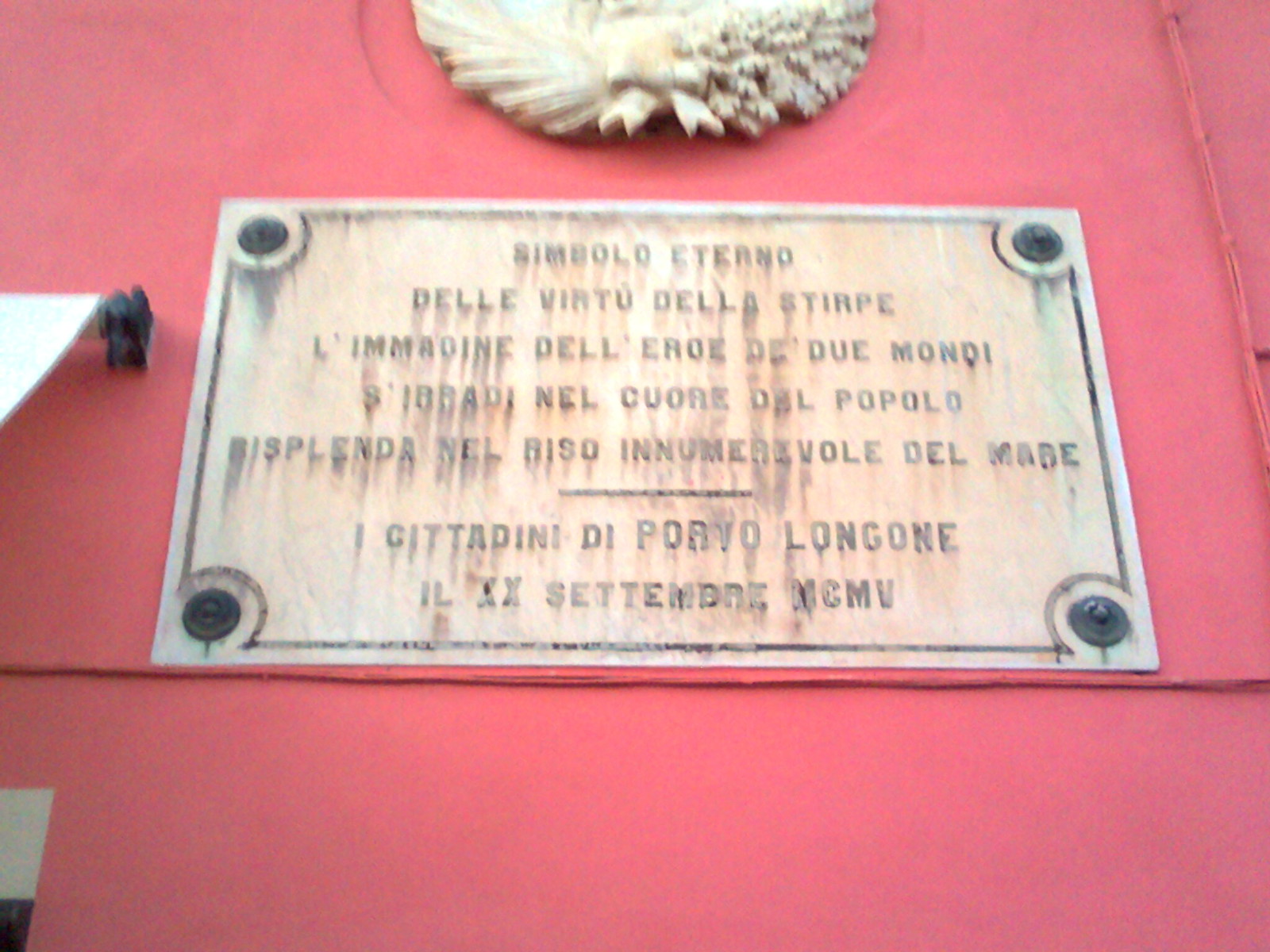The image shows a white plaque attached to a red (or pink) wall, mounted with four black screws at its corners. Above the plaque is a white plaster or clay wreath. The plaque, which appears gray and weathered with dark stains dripping from each letter, contains text in a foreign European language, possibly Italian or Spanish. The inscription starts with "SIMBOLO ETERNO" and includes several lines of text, ending with a date format resembling "IL XX SETTEMBRE MCMV." To the left of the wall is an awning, suggesting the plaque is affixed to a building.